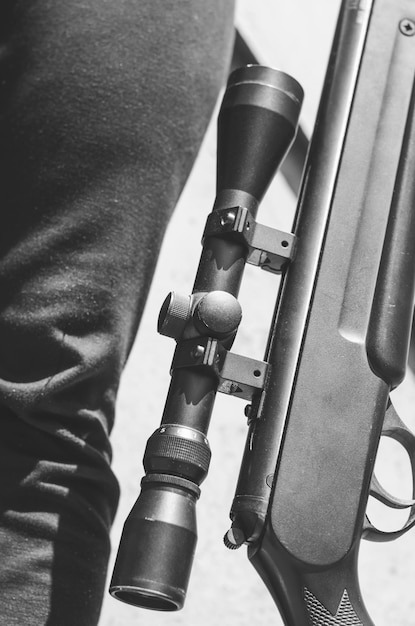This black-and-white photograph provides a detailed close-up of a rifle, emphasizing its sniper scope. The image is oriented as if viewed from the side, with the eyepiece of the scope positioned at the bottom of the frame, extending upwards along the length of the gun. The rifle appears to rest adjacent to a person, with part of their leg, likely clad in black or gray pants, visible on the left side of the image. The scope itself is notably prominent and long, extending about halfway down the neck of the rifle. The gun has a dark, textured finish with visible grip design on the handle, adding to its rugged appearance. A bolt is noticeable at the top of the rifle, securing it together. The background is a simple, nondescript gray, ensuring the focus remains on the rifle and its intricate details.